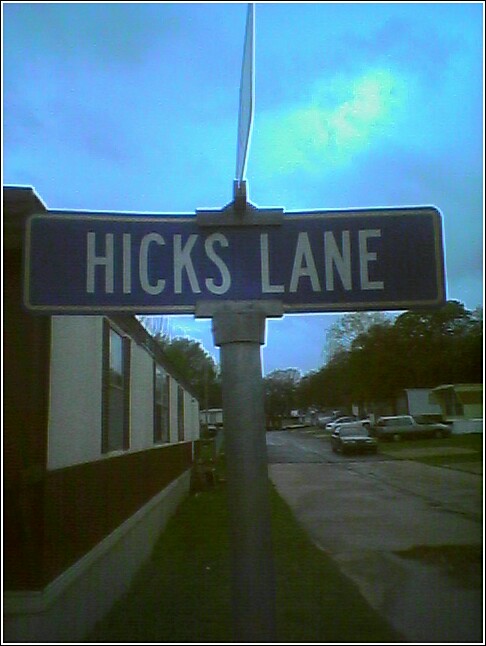The image depicts a dimly lit scene of a trailer park during daylight, characterized by a blue sky marred with clouds. Central to the image is a street sign reading "Hicks Lane," crafted in dark blue with a white border and rounded corners, and mounted on a metal pole. To the left, a large white mobile home with dark trim and two visible windows is partially in view, contrasting against its concrete base. The narrow two-lane road beside the sign stretches into the background, bordered by a small patch of grass and leading deeper into the trailer park. Numerous other trailers and various vehicles, including a car parked near the sign, are scattered throughout, underscoring a well-inhabited community. The overall darkness of the image, possibly due to low saturation or lighting, lends an aged and somber ambiance to the scene.